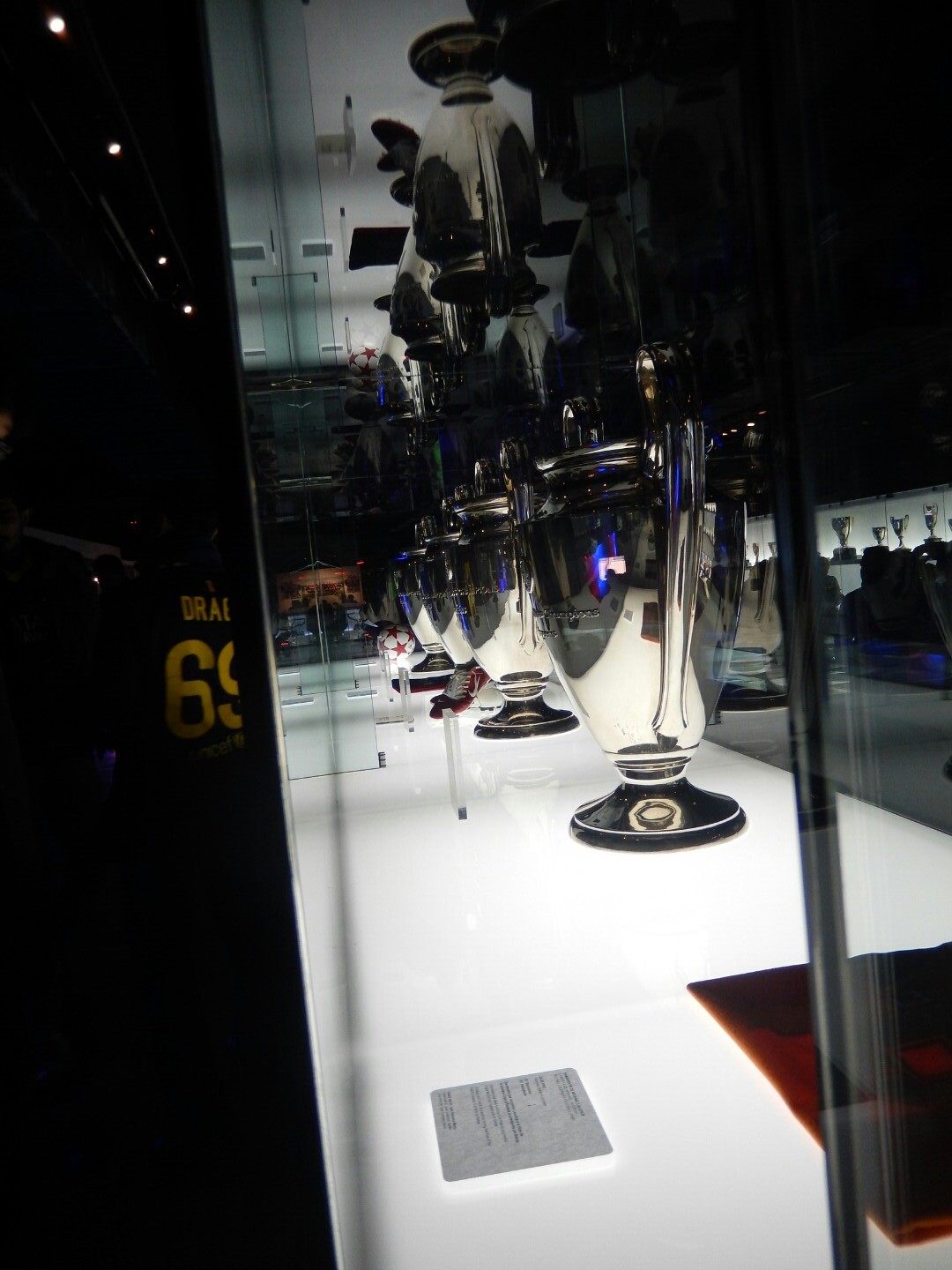The image depicts a brightly lit trophy case showcasing a collection of gleaming, silver-colored cup trophies, each adorned with elaborate handles. The base of the case is white, illuminating the trophies from below, while the top is lit, casting a clear light throughout the display. The case itself is framed in black metal and encased entirely in glass, providing an unobstructed view of the contents.

In the forefront, a striking red satin cloth lies flat with a placard placed upon it. Behind this, four silver cups are neatly lined up in a row, their intricate designs catching the light. A mirrored back adds depth to the display, reflecting the trophies and creating an impression of additional depth and multiplicity.

On the left side of the image, a sports jersey with the number 69, in bright yellow letters against a green background, is partially visible. The letters "DRA" are discernible above the number, though the rest of the name is cut off. Despite the otherwise dark room, the lighting within the cases ensures the trophies and jersey are prominently showcased.